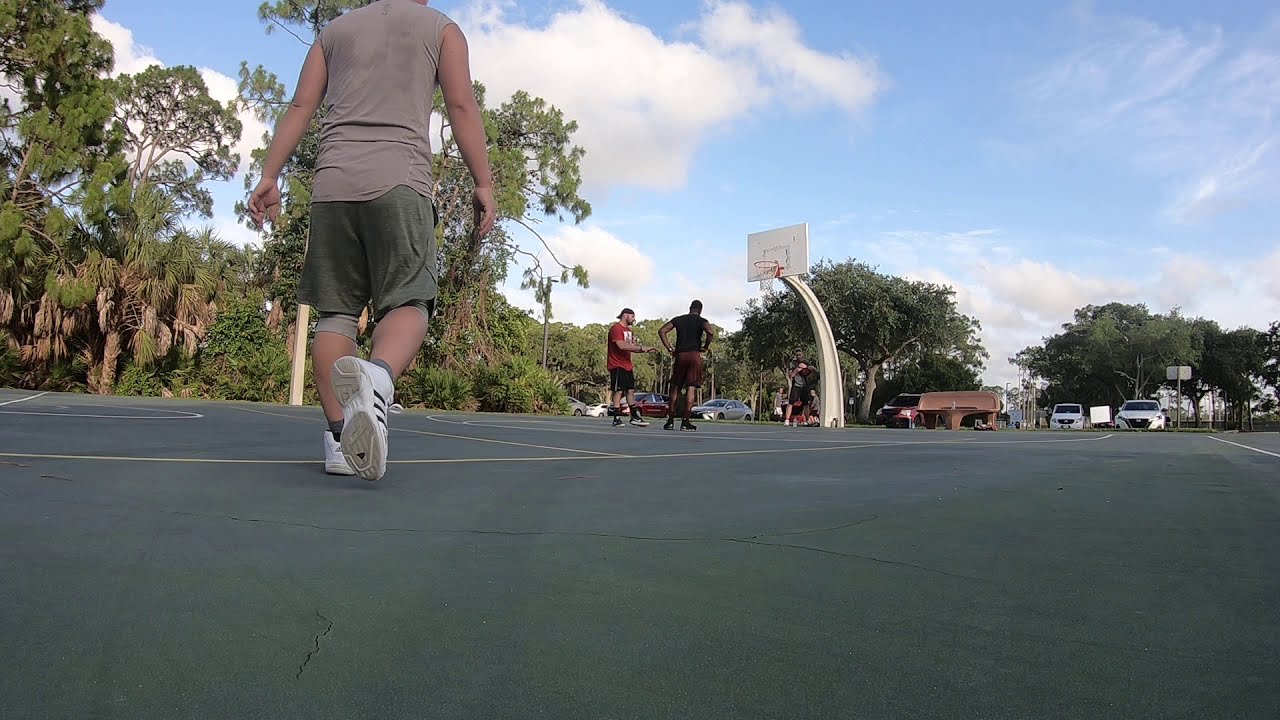This image depicts a recreational basketball scene at a park. In the foreground, a man wearing a tan sleeveless t-shirt, olive green knee-length shorts, a gray knee brace on his left leg, and white Adidas high tops with black stripes walks towards the court. To his right, two men stand near the basketball hoop; one wears a red t-shirt with white lettering, black striped shorts, and black basketball shoes, while the other sports a black t-shirt, cranberry shorts, and black basketball shoes. The court, marked with yellow and white lines on a blacktop surface, features a white basketball hoop with an orange rim. Further in the background, there's a brown bench, several parked cars in white, red, and silver colors, and a row of green-leaved trees with brown trunks. The sky above is a mix of white and sky blue clouds, captured from a low court view that emphasizes the ground and draws attention to the basketball activity unfolding at the park.